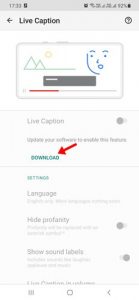This image is a somewhat blurry screenshot taken on a phone. At the top right, the battery icon displays a charge level of 92%, while the time, shown in the top left corner, reads 17:33. Beneath the time, in bold black text, the words "Live Caption" are prominently displayed with a leftward-pointing arrow beside them. Adjacent to "Live Caption" on the far right is a circle containing a question mark.

Below this header, a rectangle contains a partially drawn or perhaps video-still image. The top right corner of this image features a blue sketch of a face. On the top left, green mountains with a yellow sun are depicted. The bottom edge of this image/video displays a horizontal red bar.

Directly below this media box, there is a categorization label that reads "Live Caption," accompanied by an oval selection button to its right. Underneath this is the word "Download" in blue-green text, accented by a red arrow pointing towards it. Further down are the word "Settings" and a list of categories which include "Language," "Hide Profanity," and "Show Sound Labels."